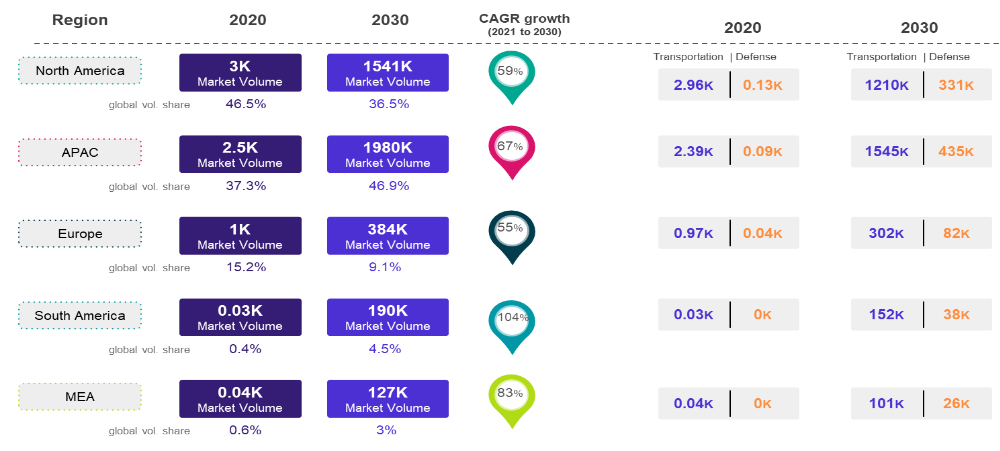The image displays an information chart with multiple columns and rows, meticulously detailing market values and growth rates across various regions over specific periods. The columns, set against a white background with black font, include: Region, 2020, 2030, CAGR Growth (2021-2030), a second 2020, and a second 2030.

The rows on the left list different regions, followed by their respective market metrics:

- **North America**: Initial market volume of 3k in 2020, projecting to 1541k in 2030, with a CAGR growth rate of 59%. Additional metrics list 2.96k, 0.13k (2020) and 1210k, 331k (2030).
- **APAC**: Starting with a market value of 2.5k in 2020, increasing to 1980k in 2030, showing a CAGR growth of 67%. Other figures include 2.39k, 0.09k (2020) and 1545k, 435k (2030).
- **Europe**: 2020 market value at 1k, growing to 384k by 2030, with a CAGR growth rate of 55%. Additional details are 0.97k, 0.04k (2020) and 302k, 82k (2030).
- **South America**: Starting at 0.03k in 2020 and reaching 190k by 2030, achieving the highest CAGR growth rate of 104%. Other stats include 0.03k, 0k (2020) and 152k, 38k (2030).
- **MEA**: Initial market value of 0.04k in 2020, expected to grow to 127k by 2030, with a CAGR growth rate of 83%. Additional figures are 0.04k, 0k (2020) and 101k, 26k (2030).

Overall, the chart provides a comprehensive overview of market dynamics and predicted growth across key global regions.